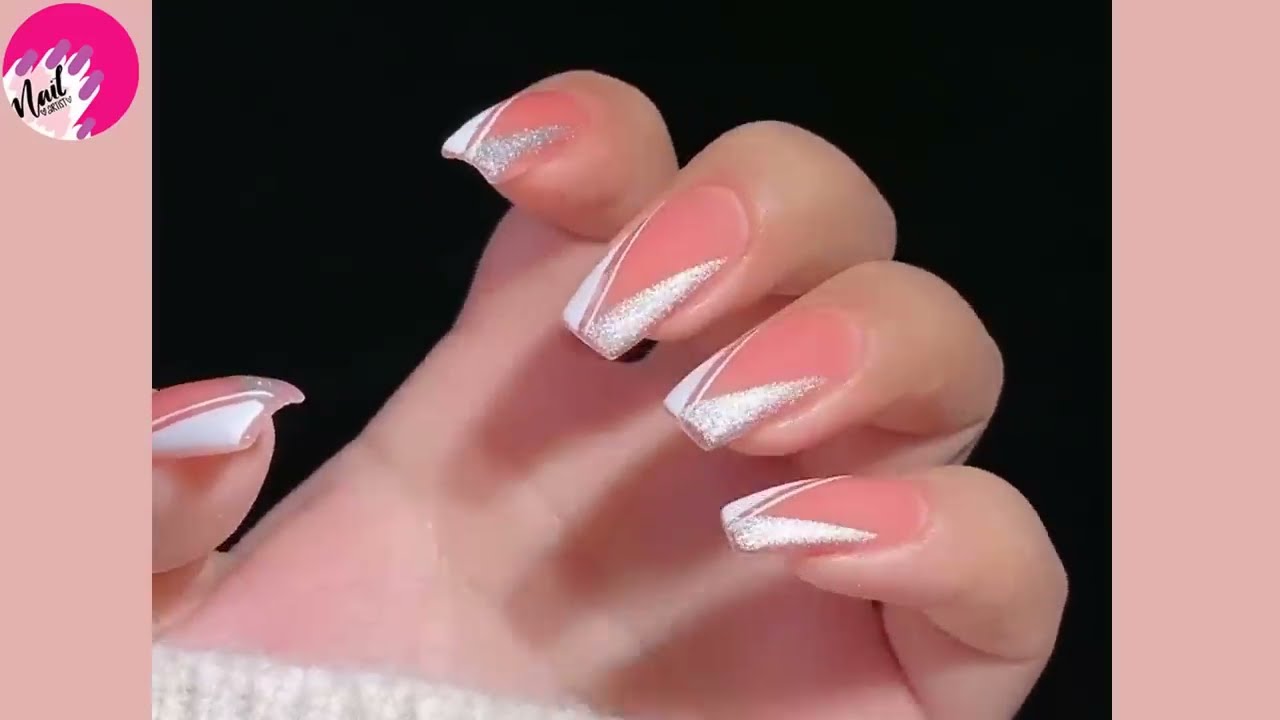The image showcases a close-up of a hand displaying intricate fingernail artwork against a divided background. The left and right sides of the image feature pale pink vertical stripes, creating a framed effect. On the left pink block, there is a dark pink circle containing an abstract drawing of a lighter-colored hand with dark purple fingernails, and the word "NAIL" written in black cursive over it. 

The central focus of the image is a human hand, prominently displayed against a black background. The hand, shown palm-up and slightly blurred, adopts a claw-like pose with fingers curved to showcase the manicure. The fingernails are styled in a block French manicure, colored pink with white and silver glitter accents forming a reverse V pattern at the tips. This design gives the appearance of pointed claws. The thumb, situated on the left side of the image, also bears the same decorative pattern. Additionally, at the base of the hand, one can discern the edge of a gray knit sweater.